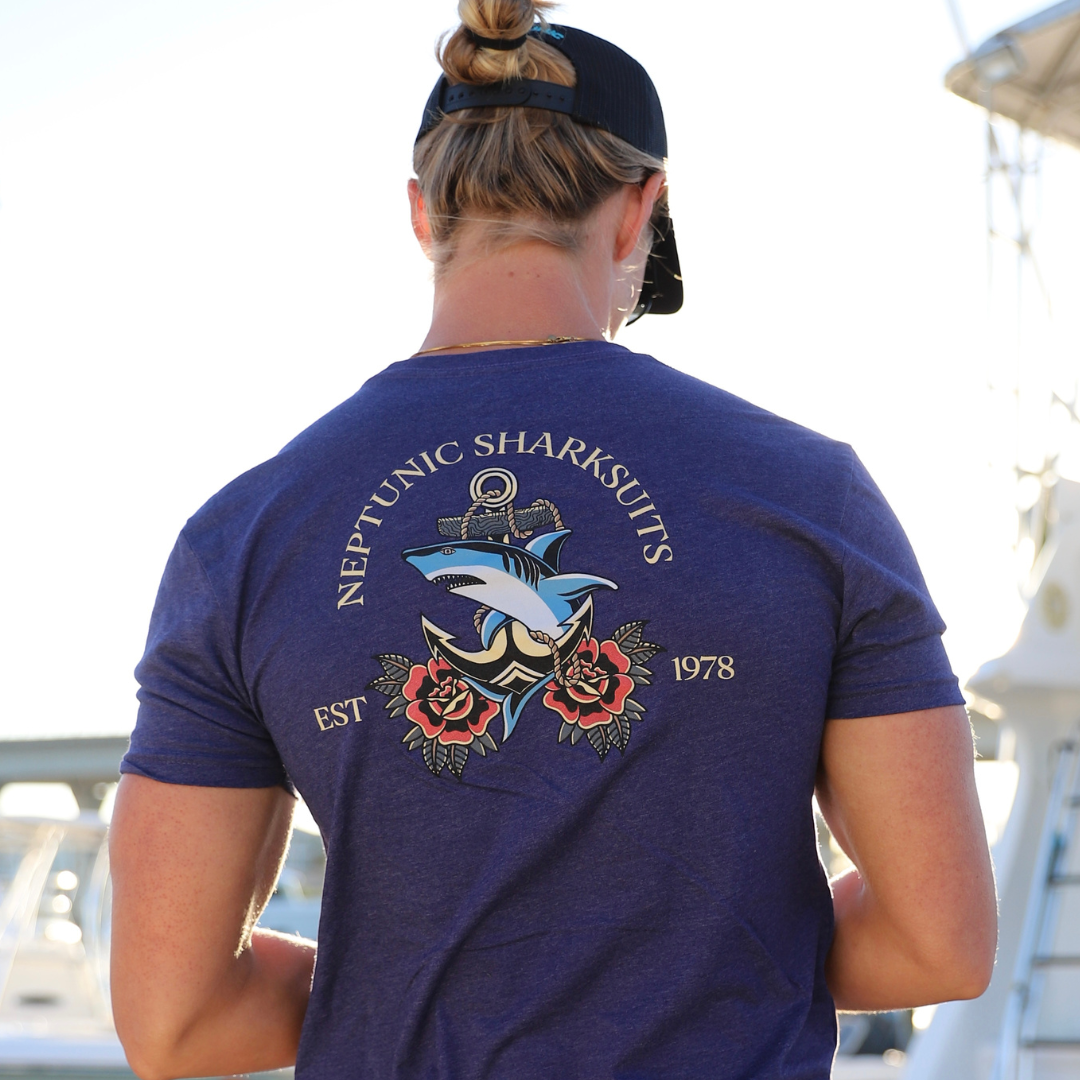In the image, we see the back of a person standing, with their entire upper body and head visible. The individual has long, medium-blonde hair styled in a bun or ponytail, held with a black hair tie. They are wearing a black hat, and their ears are adorned with earrings. The person's skin is white Caucasian, and they possess a muscular build, indicating broad shoulders and defined upper arms.

The person is clothed in a blue or purple t-shirt with a distinctive design on the back. This design features an animated blue shark entangled with a ship anchor. Surrounding the anchor are two red flowers with dark green leaves. Above this image, the text "Neptunic Shark Suits" is prominently displayed, followed by "EST 1978" positioned on either side of the anchor. The overall scene suggests a beach setting.